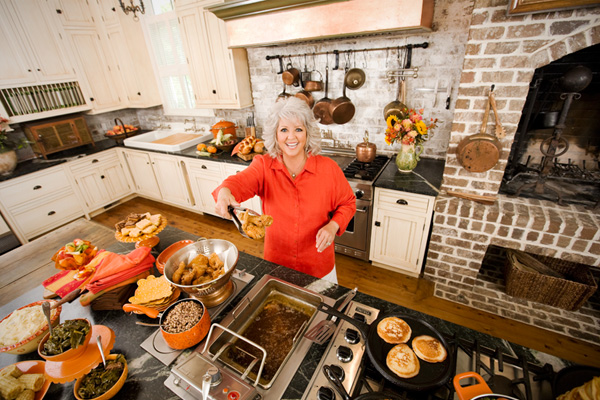This highly detailed photograph captures celebrity chef Paula Deen in her kitchen, engaged in her signature cooking activities. She stands at the center of the image, smiling warmly at the camera, dressed in a vibrant orange shirt. Her kitchen is a charming mix of rustic and functional elements, with white cabinetry and a wooden floor. Directly in front of Paula is a spacious kitchen island, adorned with numerous food items, prominently featuring fried chicken and pancakes sizzling on a grill. Paula holds a spatula in her hand, poised to continue her culinary artistry.

The background reveals a well-equipped kitchen with brass pots hanging on a brick wall, lending a cozy, homely touch. Adjacent to her, a brick fireplace adds to the kitchen's warmth and charm. There are various cooking pots on the stovetop and a collection of utensils hanging from the wall, showcasing a kitchen ready for any cooking endeavor. This photo, likely intended for promotional purposes or a recipe showcase, encapsulates the essence of Paula Deen’s culinary style and inviting kitchen atmosphere.